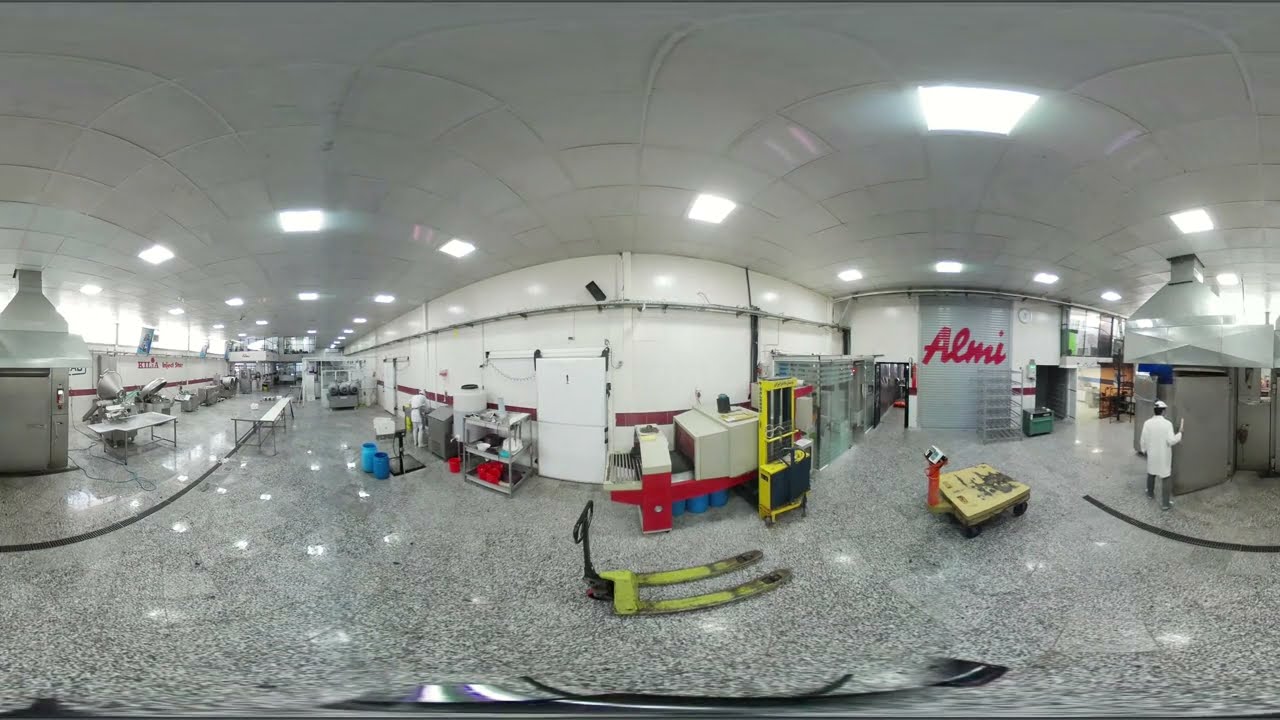The image depicts a spacious warehouse or factory interior with gray, speckled, marble-finished floors and shiny, reflective lights on the white, square-patterned ceiling. On the left side of the image, there is a prominent chrome or stainless steel door and a series of tables and shelving units that hold various items. Two blue buckets, a black stand, and additional shelving can also be seen extending towards the right.

In the central area, a greenish-colored forklift stands amidst various tools and equipment in red, white, and yellow. A small pallet jack is positioned prominently in the middle, while a nearby scale is visible towards the right. Towards the back of the image, there are boxes, barrels, and pallet movers. Above, the brand name ALMI, written in cursive red lettering, is displayed on a gray sliding door.

On the far right, a man in a white lab coat is seen opening a large stainless steel door to what could be a freezer or storage shed, possibly indicating a food processing or production facility. Next to him, there appears to be an x-ray machine or scanner, similar to those found at airports, situated beside a yellow tool. The overall layout, combined with the various pieces of industrial equipment scattered throughout, suggests an organized and efficiently designed workspace for manufacturing or processing activities.